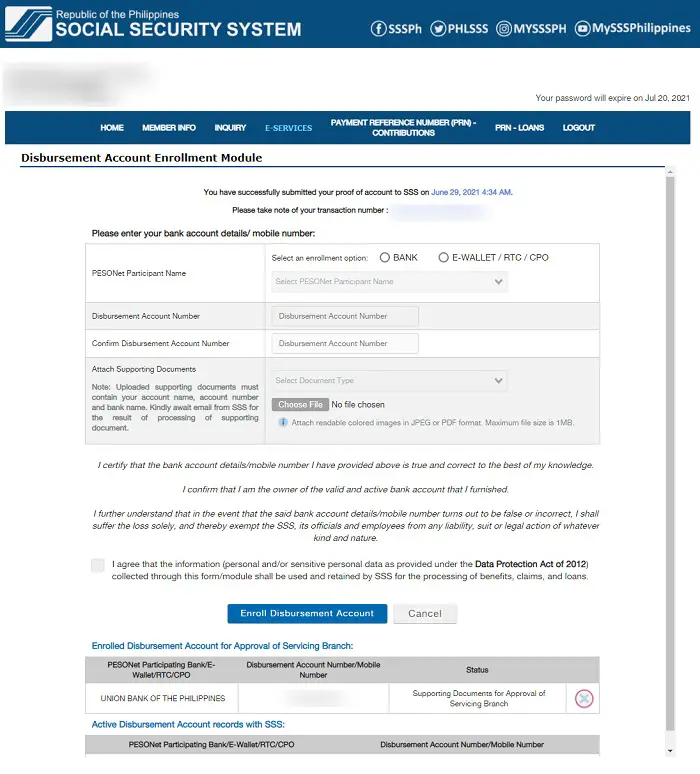The image captures a screenshot from the official Republic of the Philippines Social Security System (SSS) online portal. In the upper left-hand corner, the SSS logo is prominently displayed alongside a text indicating the organization. To its right, a row of social media icons is aligned horizontally, including a Facebook logo labeled "SSSPH," a Twitter symbol labeled "PHLSSS," an Instagram icon labeled "MYSSSPH," and a YouTube logo also labeled "MYSSSPH."

Beneath this social media section, on the right side of the screenshot, there is a notification stating, "Your password will expire on July 20, 2021." Below this notification, various navigational tabs are visible, allowing users to access different sections of the SSS portal. The tabs are arranged from left to right and are labeled: Home, Member Info, Inquiry, eServices, Payment Reference Number, PRN Contributions, PRN Loans, and Logout.

Further down, another section titled "Disbursement Account Enrollment Module" is displayed. Below it, there is a confirmation message stating, "You have successfully submitted your proof of account to SSS on June 29, 2021 at 4:34 AM. Please take note of your transaction number." Adjacent to this message, on the right side, there is an area that has been intentionally blurred, presumably to obscure sensitive information.

The meticulous arrangement and detailed information provided in this screenshot underscore the functionality and security measures of the SSS online portal.